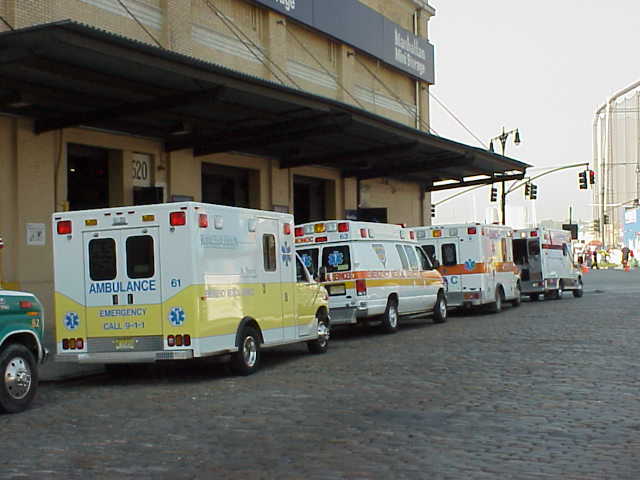This photograph captures a vintage scene, possibly from the 80s or 90s, depicting a lineup of several ambulances parked along a cobblestone street outside a yellow building adorned with large garage doors. The building, which might be a hospital, displays the address "520" and features a sign reading "Manhattan" above the garages. The street is rocky and dark grey, adding to the old-fashioned feel of the image. There are four prominently visible ambulances, each distinct in design and coloration: a mix of white with green, yellow, yellow-orange, and red stripes. The ambulances vary in size and shape, including one box-shaped vehicle clearly marked with "AMBULANCE" in blue letters and an emergency call number "9-1-1." A traffic light and streetlamp are visible, and the bright, clear sky reinforces that it’s daylight. The location and style suggest it might be in a foreign country, adding an extra layer of intrigue to the photograph.